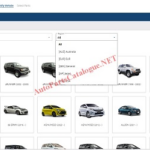The image is a blurry screenshot of questionable quality, rendering all text illegible. At the top, there is a dark blue border with an unreadable light gray caption in the left corner, likely consisting of two words. Underneath the blue border is a gray section, followed by a predominantly white background. This background showcases several cars in what appears to be a gallery.

In the center row, the vehicles include a small gray sports car, a bright taxi-yellow SUV, a white SUV, and a blue sports car on the far right. The bottom row of cars is mostly cut off, revealing only the tops of the roofs. Additionally, the row above the center is partially obscured by an unidentifiable drop-down menu. A faint pink diagonal watermark of the website address is barely visible, ending with ".net".